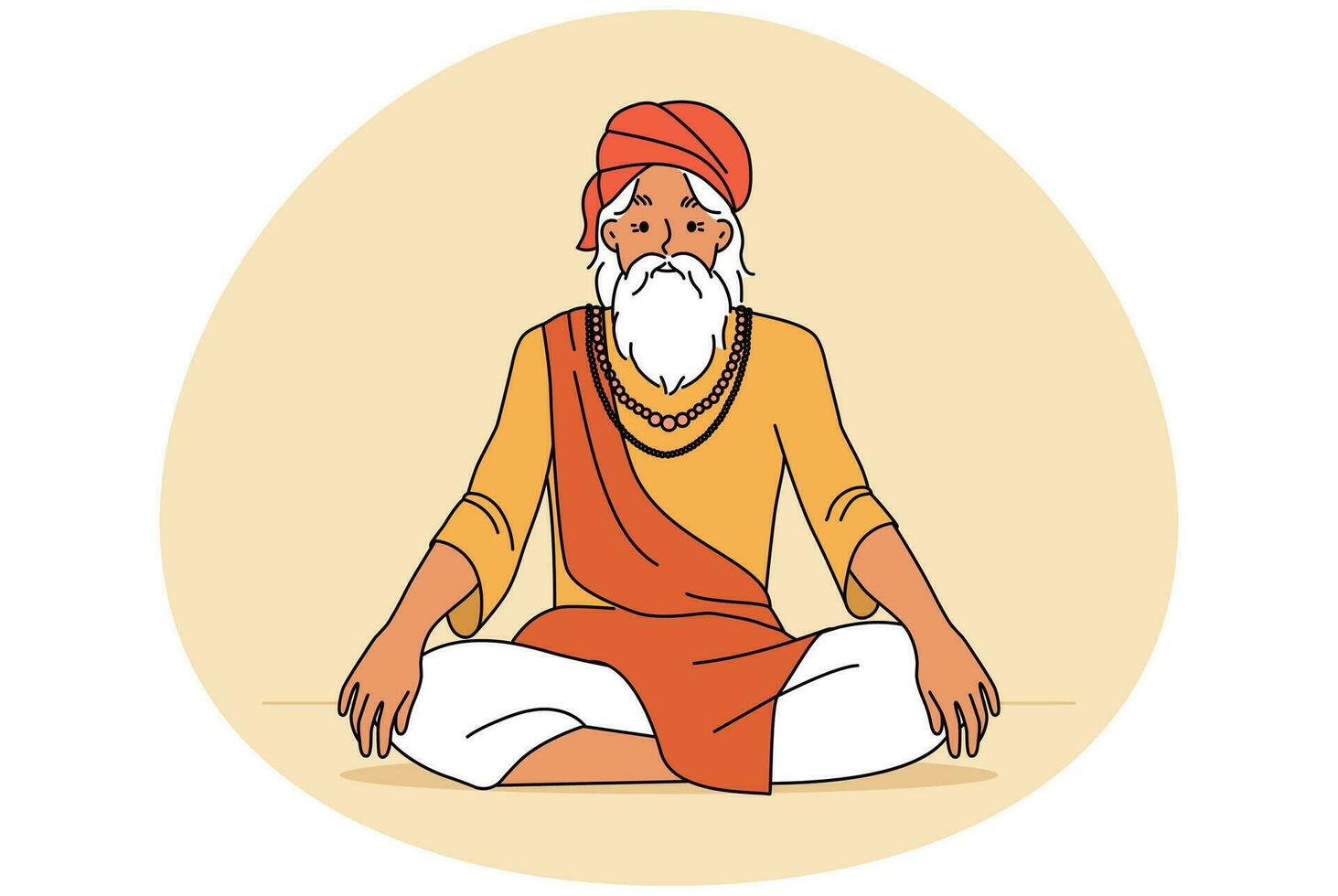The image depicts a detailed drawing of a meditative holy man, presumably from Indian culture, seated cross-legged against a beige, oval-shaped background. He has a youthful yet wise appearance with a long, white beard, white mustache, and white hair. Adorning his head is an orange turban that matches the orange sash draped around his shoulders and body. He wears a golden yellow shirt with baggy sleeves that extend just past the elbows, and loose white pants. His hands rest on his knees in a balanced and serene posture. Around his neck, he wears multiple necklaces: one made of golden beads and another resembling a black lace or chain. His dark skin contrasts with the light hues of his clothing and the beige backdrop. The man's figure casts gentle shadows, adding a sense of depth to the composition and emphasizing his tranquil and spiritual demeanor.